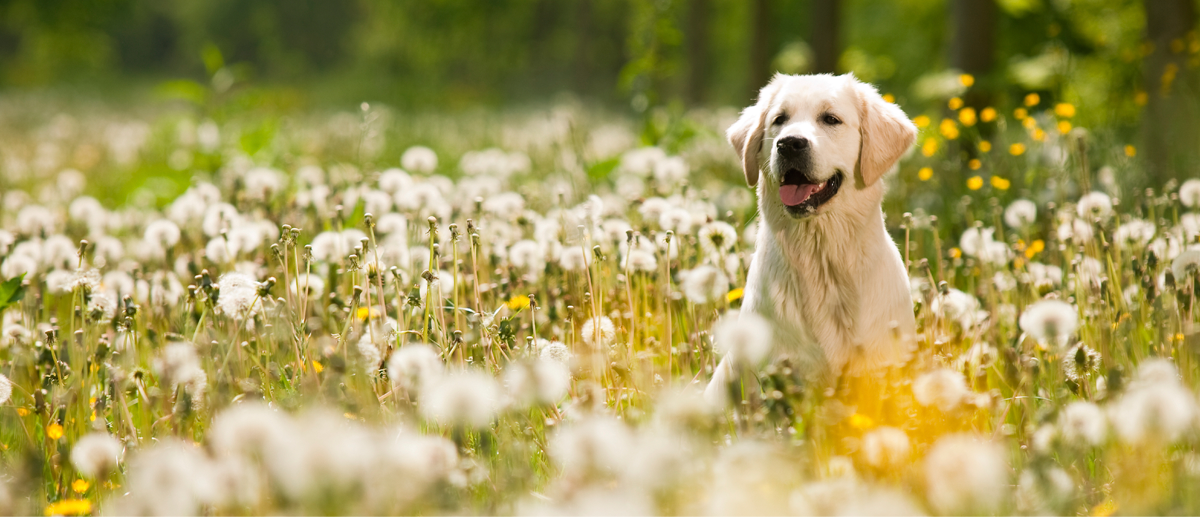This professional photograph captures a lively golden retriever in a blooming field of dandelions and other wildflowers. Though positioned to the right side of the frame, the creamy white golden retriever is the unequivocal focal point of the image. With his mouth open and pink tongue hanging out, the dog gazes joyfully into the distance, embodying a sense of contentment and happiness. His floppy ears drape forward, enhancing his playful demeanor. The lush green foliage around him is dotted with white and tan dandelions—the kind you blow—as well as an array of bright yellow flowers. The blurred background includes a hint of tree trunks and dense greenery, suggesting an outdoor springtime setting bathed in sunlight, which further accentuates the vibrancy of the scene.